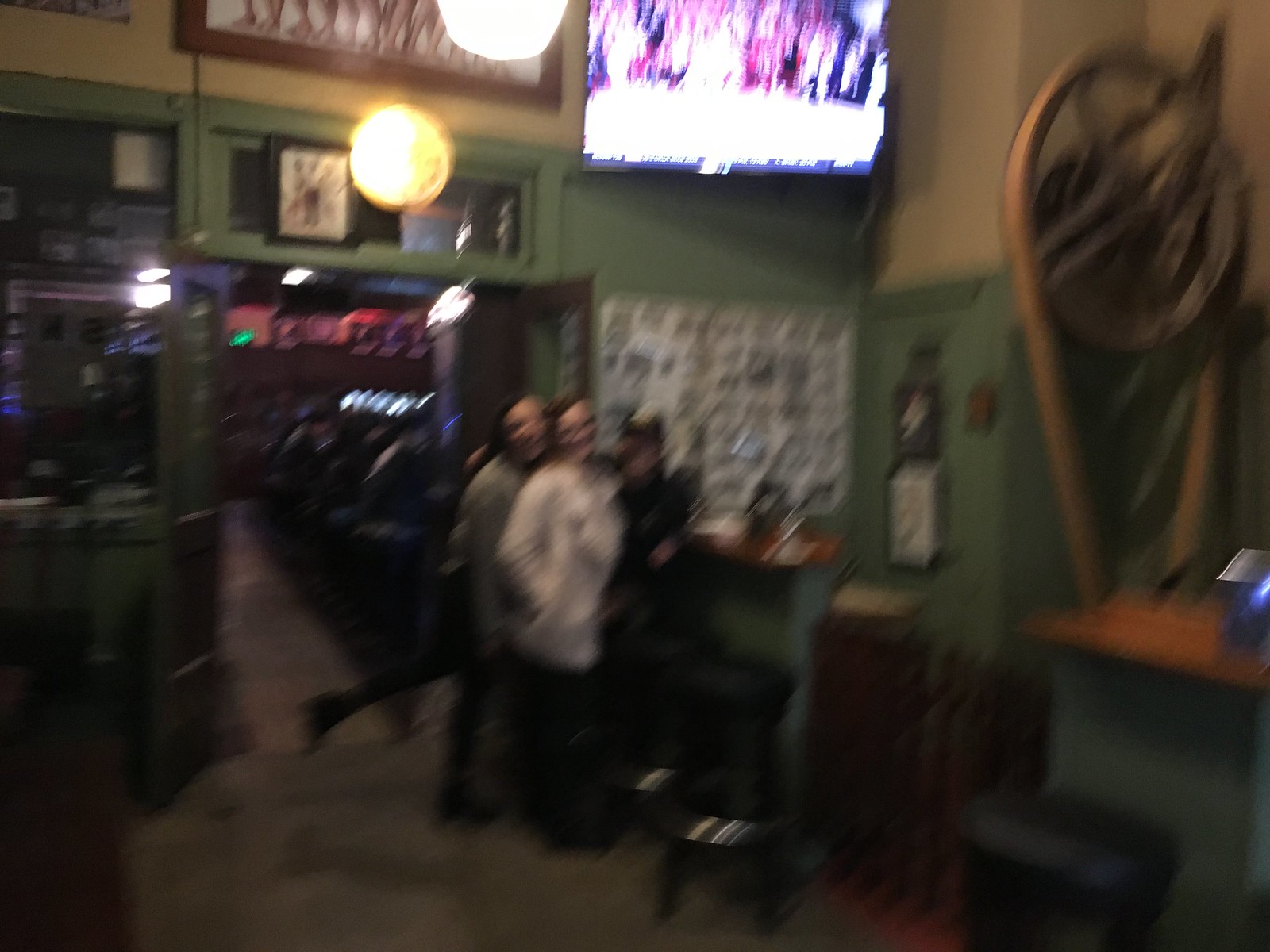In the very blurry photograph of a bar's interior, three people are huddled closely together for a group photo, two women and one man. The woman on the left, wearing a green shirt, is stretching her leg out backward. The second woman is dressed in a white sweater or jacket, and the man is donning dark clothes along with a possible baseball cap. They are standing near a high top table with black stools, directly in front of a set of double doors that seem to lead to another part of the bar. Visible elements include green and yellow walls, various signs, pictures, and a TV that is on in the corner, suggesting it might be a sports bar. There's a bulbous, gold-colored hanging light and a clock above the door, which opens into a larger room illuminated by further lights. Despite the significant blurriness making it hard to discern precise details, these key elements are discernible.